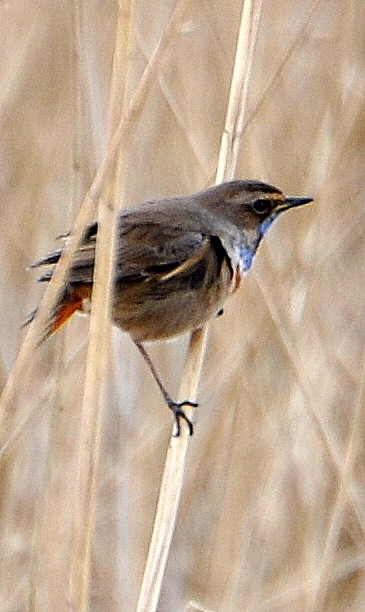This portrait-mode nature photograph captures a small, chubby bird in sharp focus against a blurred background of dry grass, reeds, and straw. The bird, perched on a diagonally angled twig, has a slender black beak facing to the right. Its overall plumage is a mix of dark brown and grayish tones, with distinctive blue tints on its neck and chest, and a touch of red on its tail feathers. The bird's black legs grip the light brown twig securely, demonstrating its delicate stance in a serene natural setting. The image beautifully highlights the bird's detailed and varied coloration.